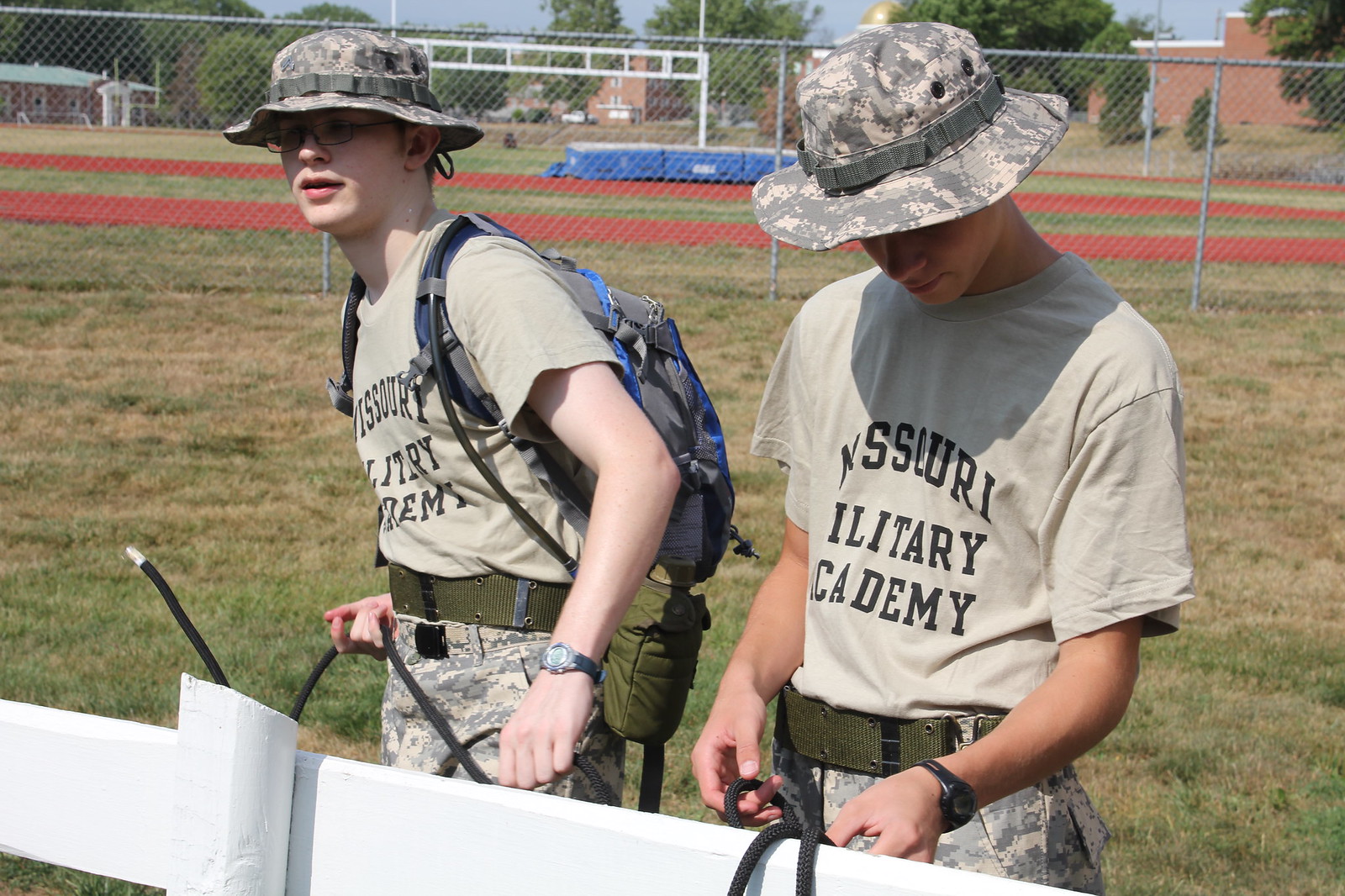The rectangular photograph captures a vivid outdoor scene at the Missouri Military Academy, featuring two young cadets, likely around 15 years old, engaged in an activity by a white plank fence. Both cadets are adorned in camouflaged bucket hats, olive-colored t-shirts emblazoned with "Missouri Military Academy," thick green woven belts, and khaki pants. One cadet wears glasses and a watch, while the other sports a backpack and possibly a canteen holster. The cadet on the left is seen meticulously tying a green rope to the fence, while the cadet on the right holds a similar green rope. Behind them stretches a grassy field, bordered by a chain-link fence that encloses what appears to be a running track, a football field goal, and expansive grounds leading to brick buildings and trees in the distance. The scene is bathed in bright natural sunlight, enhancing the vivid details of the cadets' activity and their uniforms.